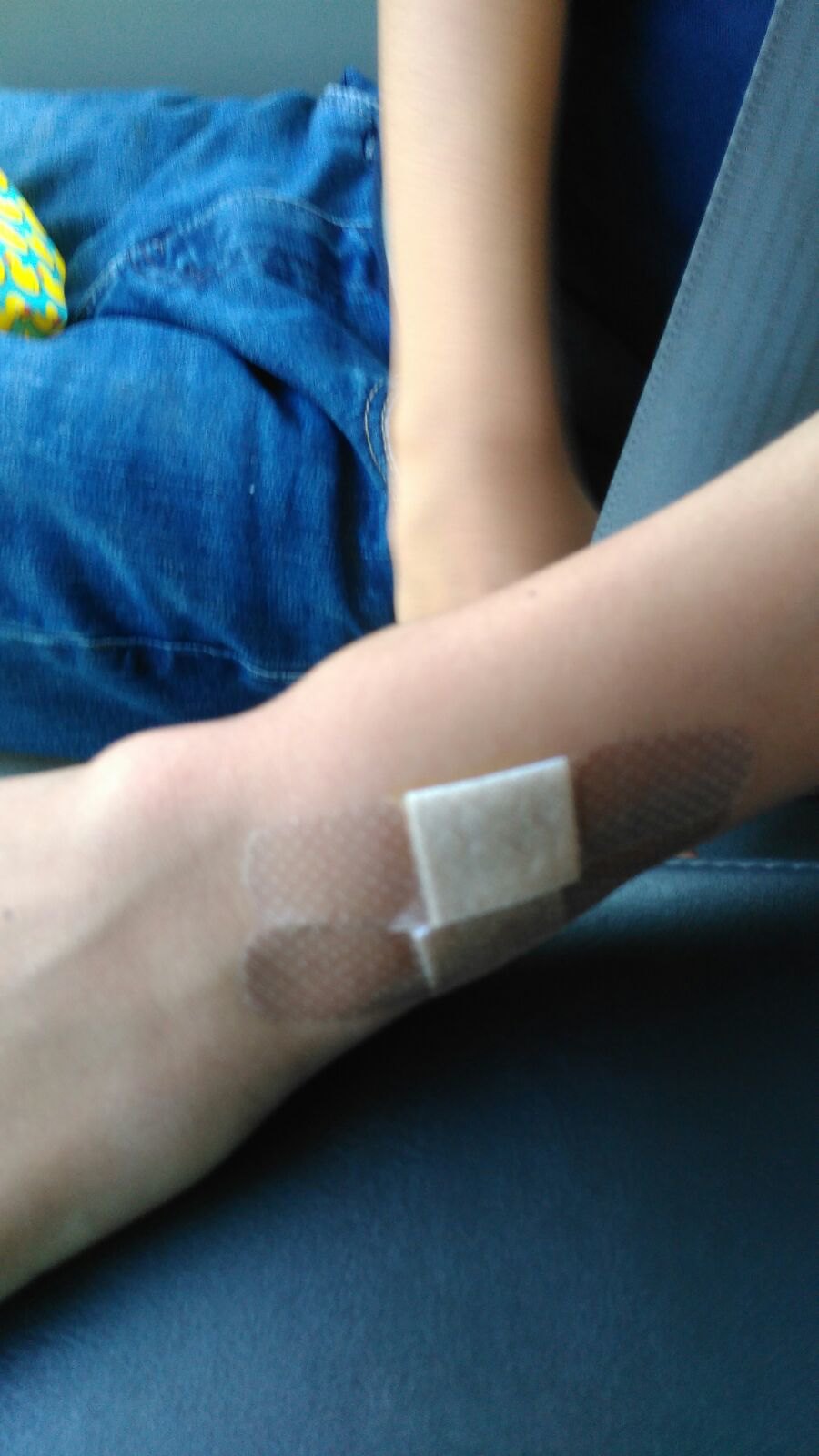In this slightly blurry, color photograph taken indoors, a close-up view captures a Caucasian child's wrist and hand positioned diagonally from right to left. The back of the child's wrist features two stacked band-aids, each brown with white dots and a white pad in the center, covering what appears to be a slight swelling. The child is seated, presumably in a car's passenger seat, as indicated by the visible gray seatbelt across their lap and torso. They are dressed in regular blue jeans and a navy t-shirt, with a green object, possibly adorned with yellow duck patterns, partially visible in their lap. The other arm, without any band-aids, rests over their lap, seemingly interacting with the seatbelt.